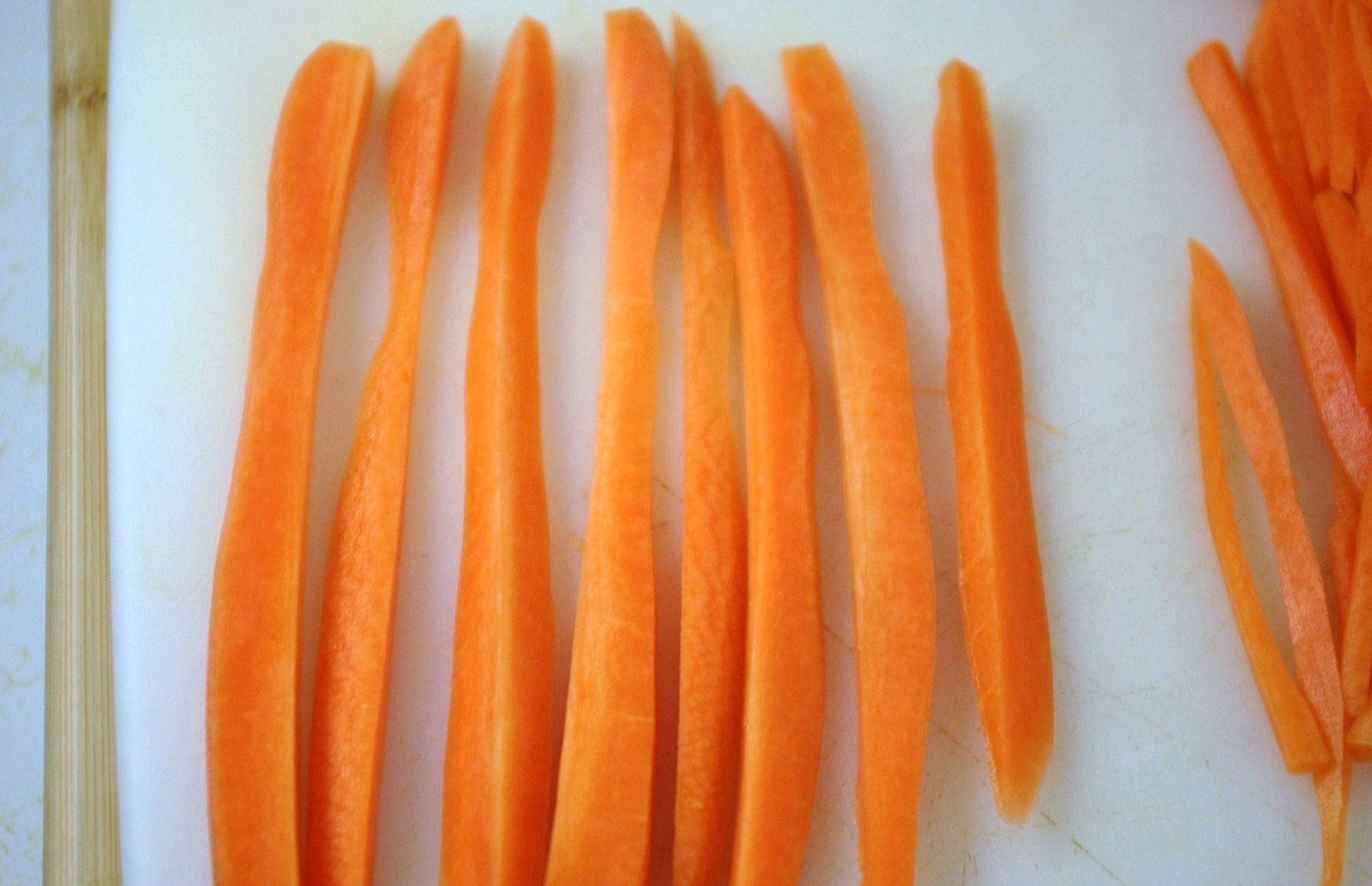This overhead photograph captures a white cutting board with a wooden border, displaying freshly cut, vibrant orange carrot slices. The cutting board, bearing numerous knife marks, rests on a white surface that may be marble or granite, characterized by subtle gold veining. On the left, a brown, wooden stick extends vertically, cropped by the edge of the image. Central to the composition, eight meticulously julienned carrot strips are arrayed in a neat row. To the right, additional, thinner carrot slices are gathered into a less ordered pile. The bright, moist appearance of the carrots suggests they have been recently prepped, likely for culinary use.